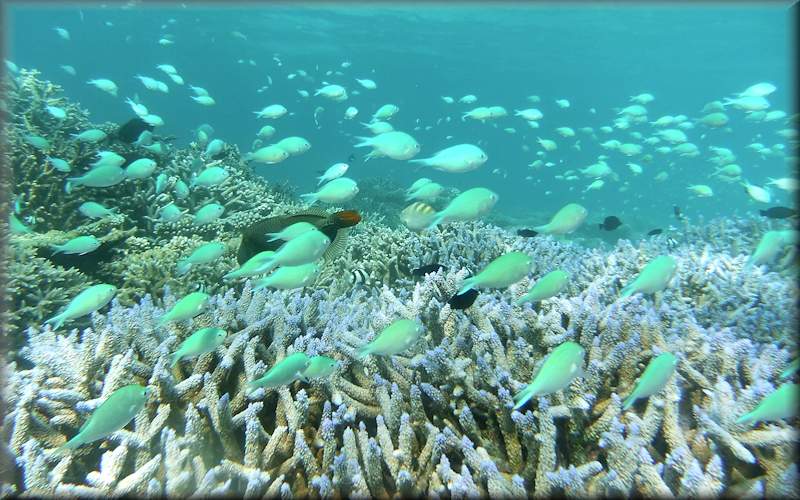This underwater photograph captures a vivid scene deep in the ocean. Along the bottom, there's an expansive coral reef displaying a symphony of light colors, primarily purples, blues, and hints of orange-red. Amidst the coral, hundreds of bright, cyan-colored fish swim predominantly from left to right, creating a mesmerizing, glowing effect against the clear, blue-green water. The fish, teardrop-shaped with pointed tails, form a cohesive school, although some can be seen swirling in different directions, adding dynamism to the scene. Hidden among the school are a few larger, darker fish, possibly groupers or puffer fish, though hard to identify with certainty. The left-hand corner of the photo features an even denser cluster of coral that extends upward. Above this vibrant underwater ecosystem, the deep blue sea provides a serene backdrop, illuminated by what seems to be late afternoon sunlight, offering excellent visibility that allows the viewer to see every detail of this bustling underwater world.